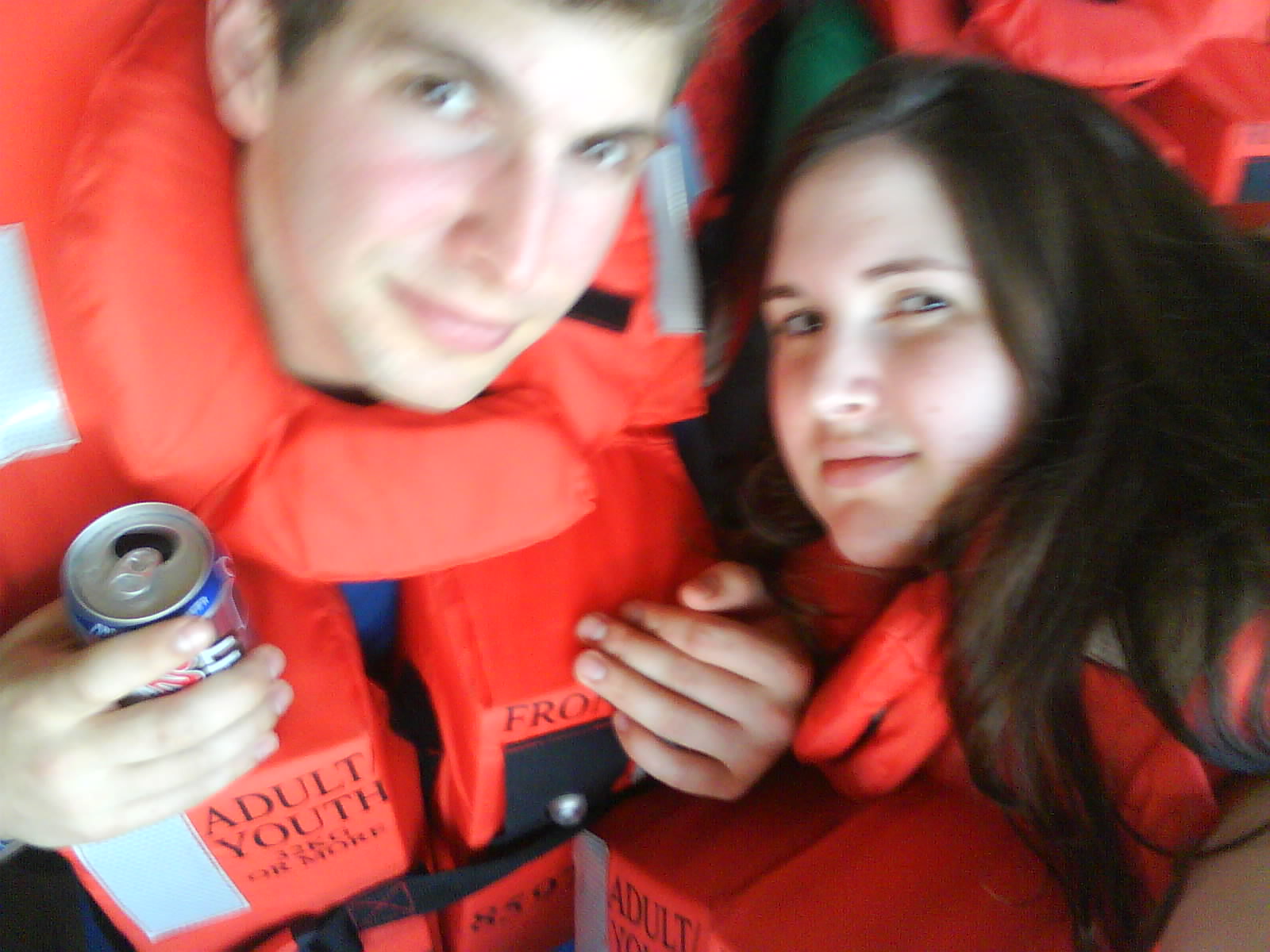In this somewhat blurry close-up photo, a young couple stands closely together, both somewhat smiling at the camera. Each person is wearing a bright orange life preserver with the label "adult youth." The man, who has short hair and a rosy complexion, holds a can of Coors Light and is looking directly at the camera. The text "32 kg or more" is also visible on his life preserver. Beside him, the woman with long, dark brown hair cascading beyond her shoulders glances towards the camera, her lips partially red. The background features an orange and green fabric, hinting at a possible outdoor or boat setting. Despite the blur, their fair complexions and attire are clearly visible, providing a vivid yet imperfect snapshot of the moment.